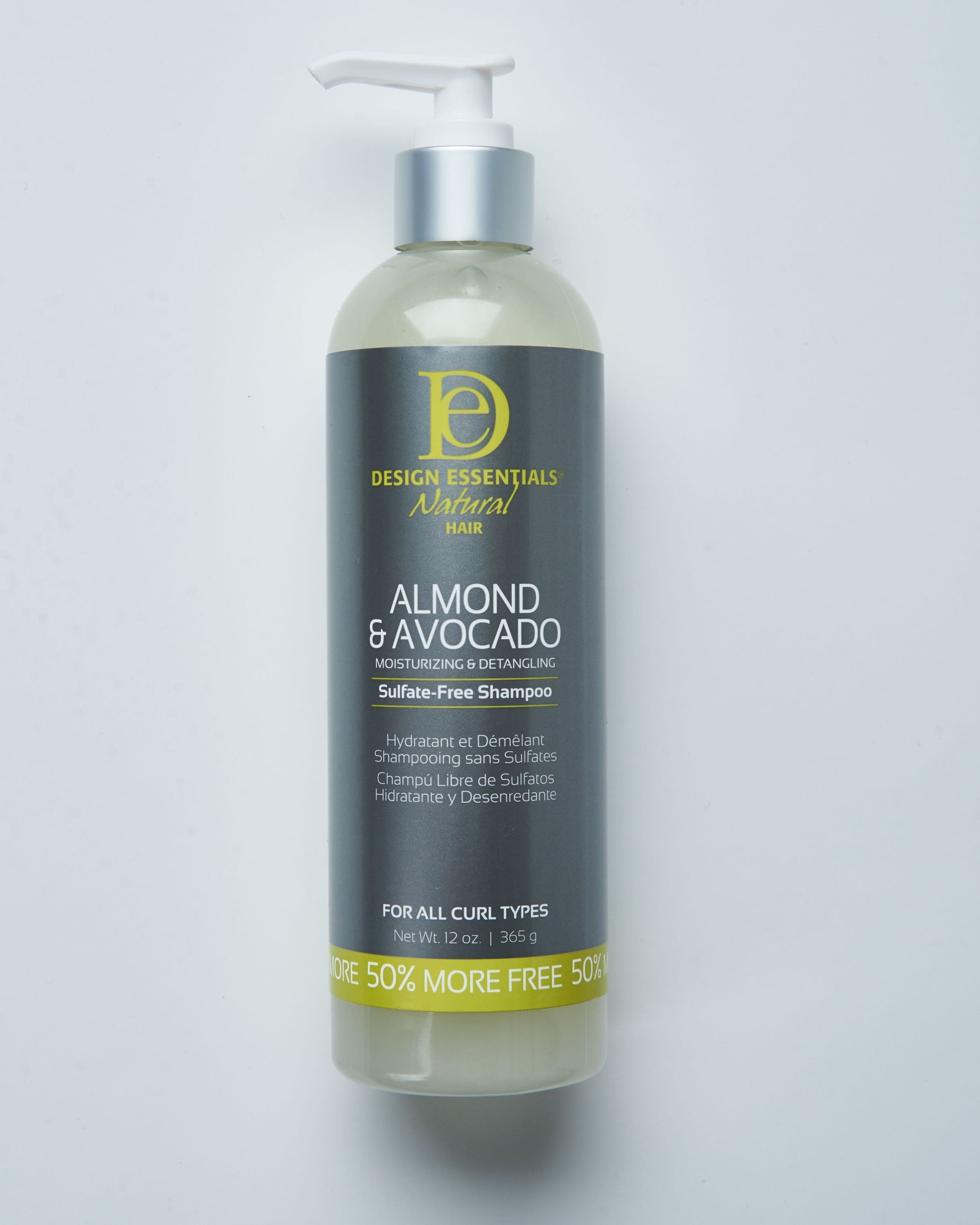This close-up indoor photograph showcases a 12-ounce (365 grams) bottle of Design Essentials Natural Hair Almond and Avocado Moisturizing and Detangling Sulfate-Free Shampoo. The bottle is centered against a grayish background, presenting a sleek and brand-new appearance. It features a white pump dispenser and a clear body filled with a creamy liquid. The wrap around the bottle is a dark gray color with mustard yellow lettering that highlights the brand name. In capital white letters, the label elaborates on the product's features: "Almond and Avocado Moisturizing and Detangling Sulfate-Free Shampoo." Additionally, it includes text in another language and mentions that it's suitable for all curl types. At the bottom, a gold background banner prominently states "50% more free." This detailed image would be ideal for online advertising or selling platforms like eBay.